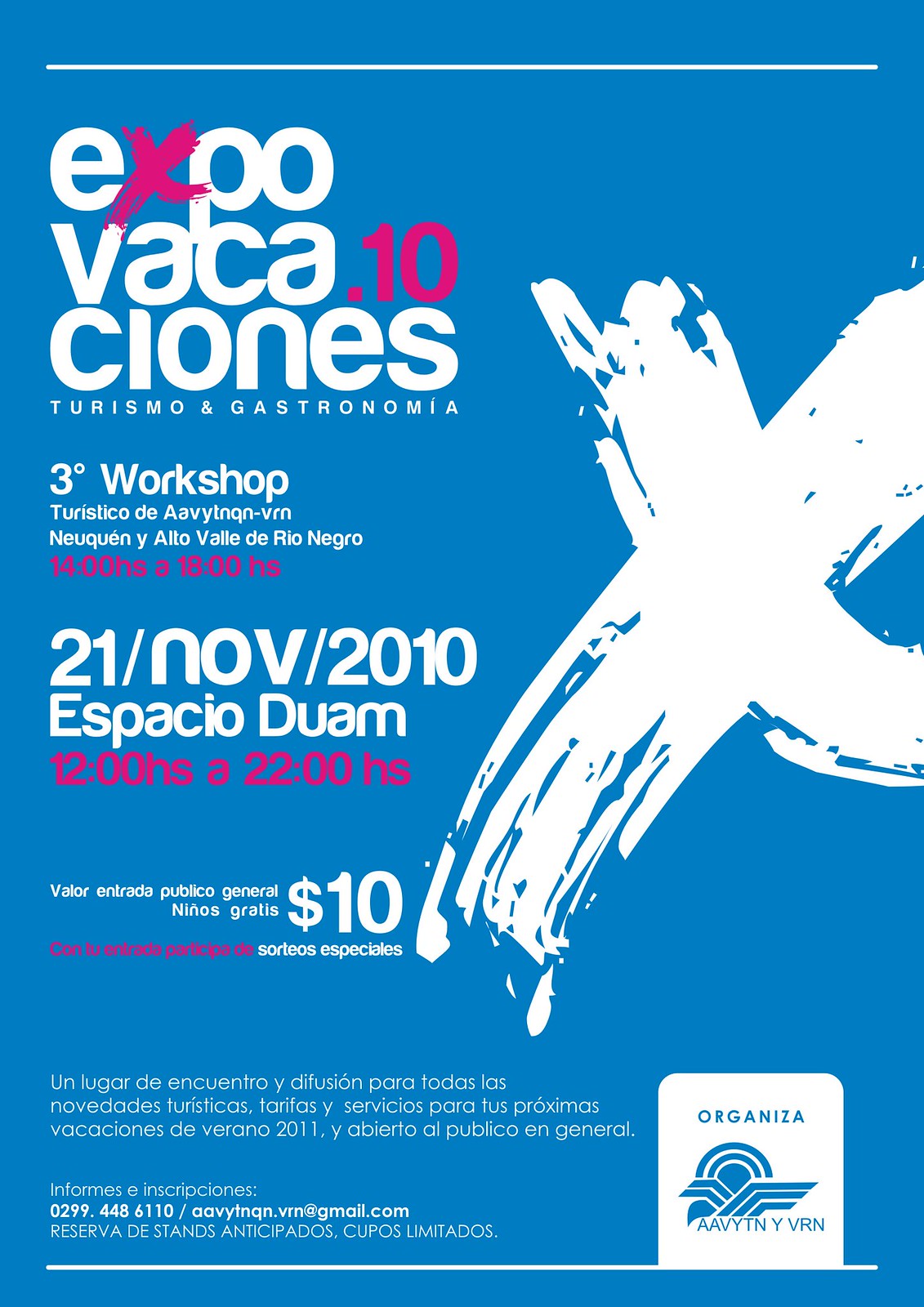The image is a vibrant blue poster predominantly featuring white text with accents of a paintbrush-like red. At the top, a white bar runs horizontally, almost spanning the poster’s width, with the text "EXPO VACA.10 CIONES." The "X" and "10" are highlighted in red, while the rest of the text remains white. Below this title, in smaller white print, it reads "Turismo and Gastronomía."

To the right of the text, a red paintbrush swirl creates a dynamic visual element. Beneath the main title, additional event details are provided, including "Three Degree Workshop in Turismo," followed by "Nequén y Alto Valle del Río Negro." 

Timings for the event are indicated in red as "14 HS - 18 HS." The date "21 NOV 2010" is displayed clearly in white, followed by "ESPACIO DUAM." Below these, another time slot reads "1200 hours - 2200 hours," also in red. Near the bottom-right corner, there are details about the organizer, denoted by "ORGANIZADO," accompanied by a logo. There's also a contact section with a phone number and email address, although these are small and difficult to decipher. The price of admission is prominently listed as "$10."

Overall, the poster provides a comprehensive overview of the "Expo Vacaciones" event in Spanish, with visual elements and detailed information designed to attract and inform potential attendees.